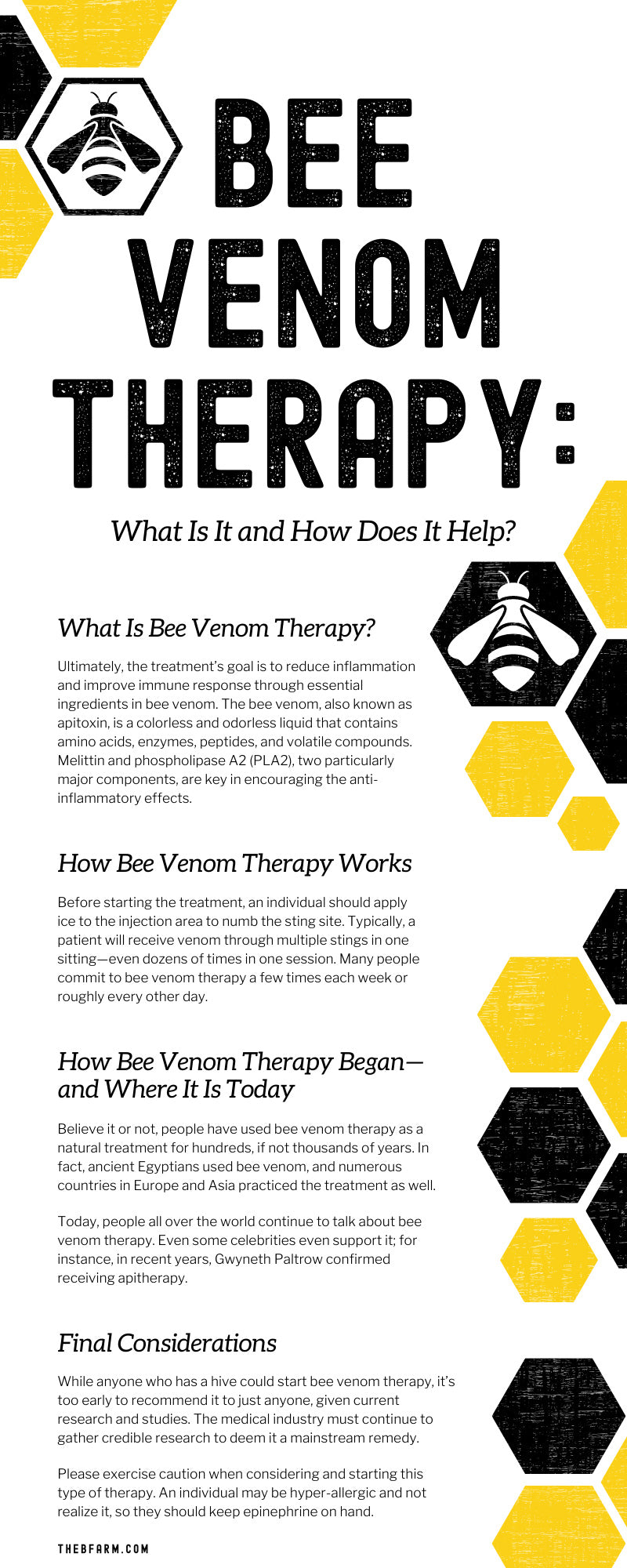The scanned image depicts an informative notice titled "Bee Venom Therapy" at the top, written in black text. The design features yellow and black hexagons scattered throughout, some of which contain a bee logo. The notice is structured into several sections, each providing detailed information about bee venom therapy. These sections include: "What is Bee Venom Therapy?" followed by a detailed paragraph; "How Bee Venom Therapy Works," accompanied by an explanation in smaller font; and "How Bee Venom Therapy Began and Where It is Today," which includes two short paragraphs. The document concludes with "Final Considerations" and additional notes. The bottom left corner of the notice includes a reference to "thebeefarm.com."